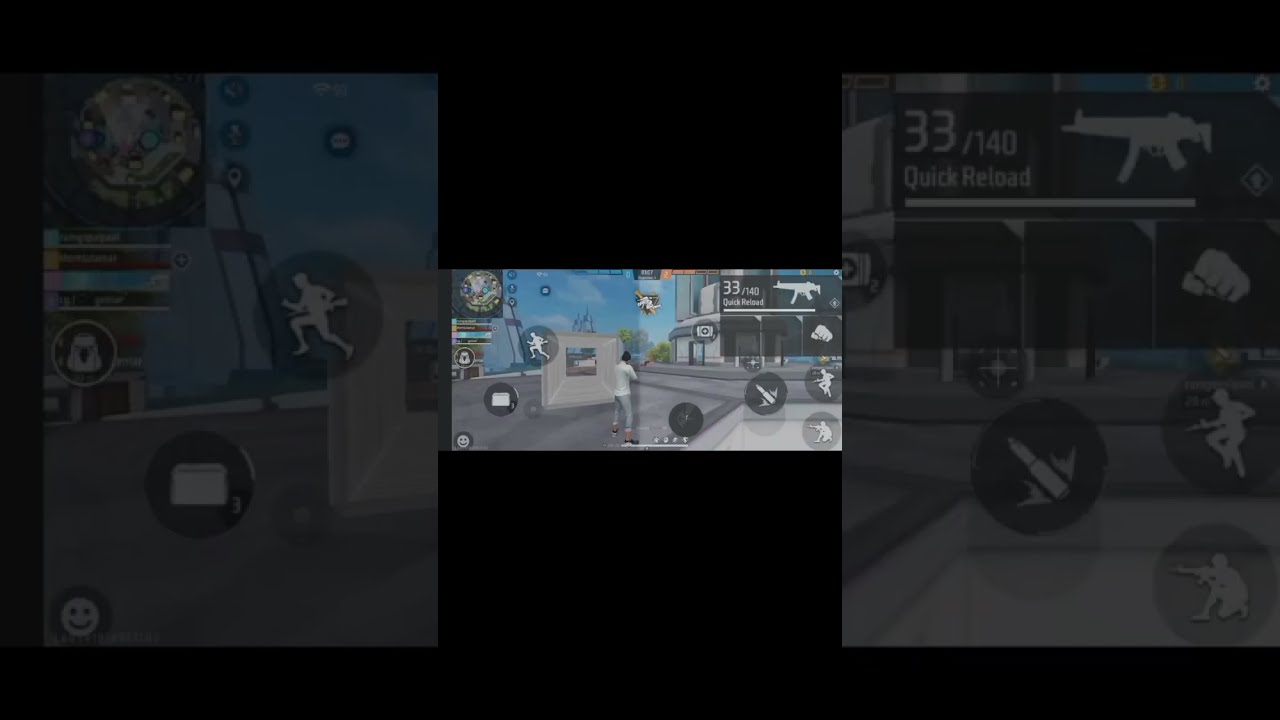The image depicts a small screenshot of a shooter video game against a black background, with the central character positioned in the center of the frame. The character, dressed in gray pants and a white sweater, is crouching and holding a rifle, aiming into what appears to be a tunnel. To the right of the character is a control panel displaying various icons, including options for missiles, a running soldier, a fist, and a crouching soldier. The top left corner features a radar, while the top right corner displays a larger assault rifle icon with an ammo count of 33 out of 140, and the words "Quick Reload." The scene shows the character hiding behind a metal box in the middle of a street, surrounded by buildings, with colors predominantly in blue, white, light blue, gray, black, and orange. The overall style suggests the game could be played on a mobile device or computer.